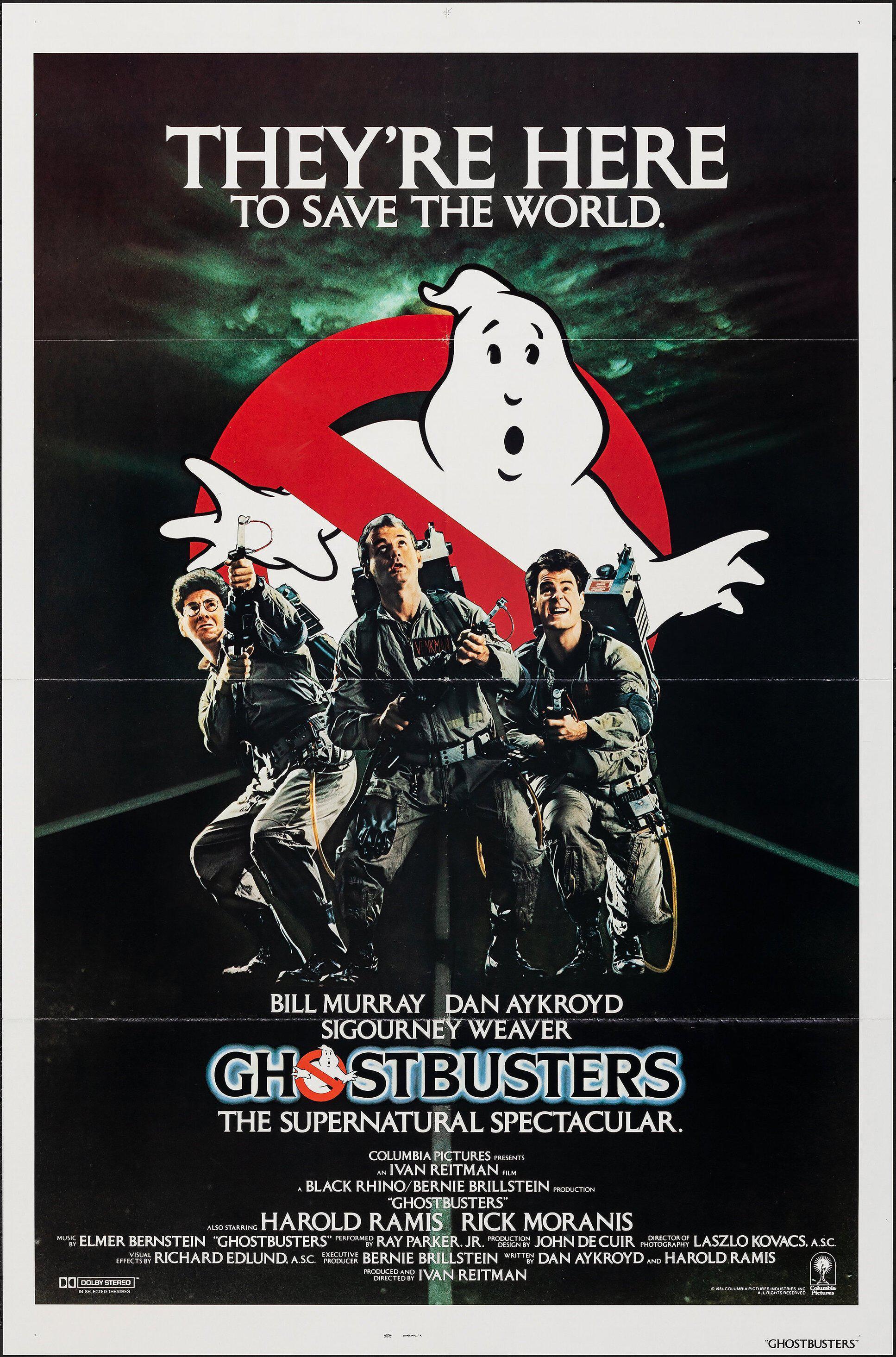This is a highly detailed movie poster for the original "Ghostbusters." The top of the poster features the tagline, "They're here to save the world," in white text. Dominating the upper section is the iconic Ghostbusters logo—a white ghost behind a red "do not" symbol. Below the logo are the four main characters: Bill Murray, Dan Aykroyd, Sigourney Weaver, and Harold Ramis, all dressed in their signature gray jumpsuits with proton packs on their backs. The poster has a striking black background with eerie green clouds emanating from behind the logo, adding a supernatural ambiance. The movie's title, "Ghostbusters," appears in bold black text with a white outline and blue shading, with the O in "Ghostbusters" ingeniously designed as the ghost logo. The tagline "The Supernatural Spectacular" follows beneath the title, accompanied by the credits listing the cast and crew involved in the film.